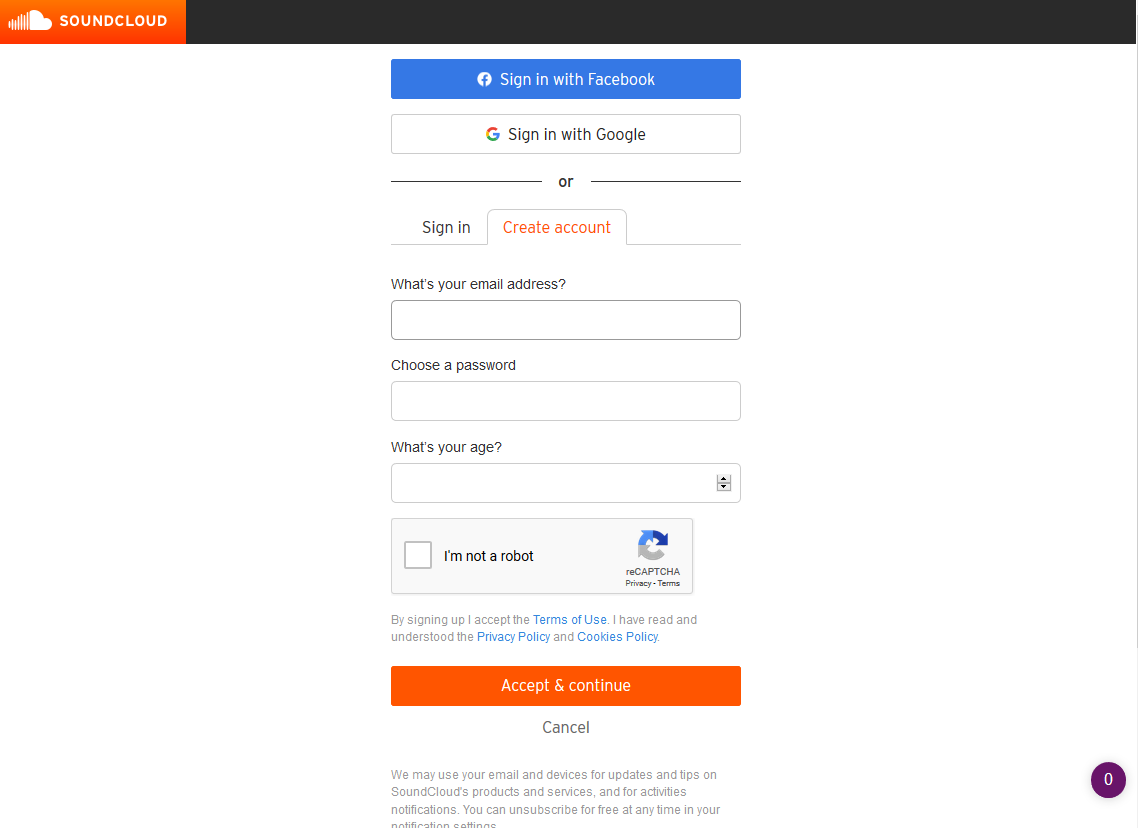Here is a detailed and cleaned-up version of the caption:

"This image is a screenshot of the desktop version of the SoundCloud website sign-in page. At the top right corner, there's an orange rectangle featuring the SoundCloud logo. Adjacent to this, the rest of the top segment of the page is a black rectangle. The background below is primarily white. 

Centered on the page is the sign-in section. At the very top, there is a prominent blue bar labeled 'Sign in with Facebook.' Immediately below, there is a white bar labeled 'Sign in with Google.' 

Under these options, the word 'or' is centered on the screen. Below the 'or', there are two tabs: 'Sign in' and 'Create account.' The 'Create account' tab is selected, so 'Create account' is highlighted in red.

The first input field asks 'What's your email address?' followed by a text box for the user to enter their email. The second input field prompts 'Choose a password,' also accompanied by a text box. The third input field asks 'What's your age?' and features a drop-down menu for selection.

Towards the bottom of the form, there is a CAPTCHA box with the CAPTCHA logo to the right and a checkbox to the left. The checkbox is labeled 'I'm not a robot.'

Directly below the CAPTCHA, there are links to the 'Terms and Conditions,' 'Privacy Policy,' and 'Cookie Policy,' which are highlighted in blue text. At the very bottom of the page, there is a large orange button labeled 'Accept and Continue,' and beneath that, centered text that reads 'Cancel.'"